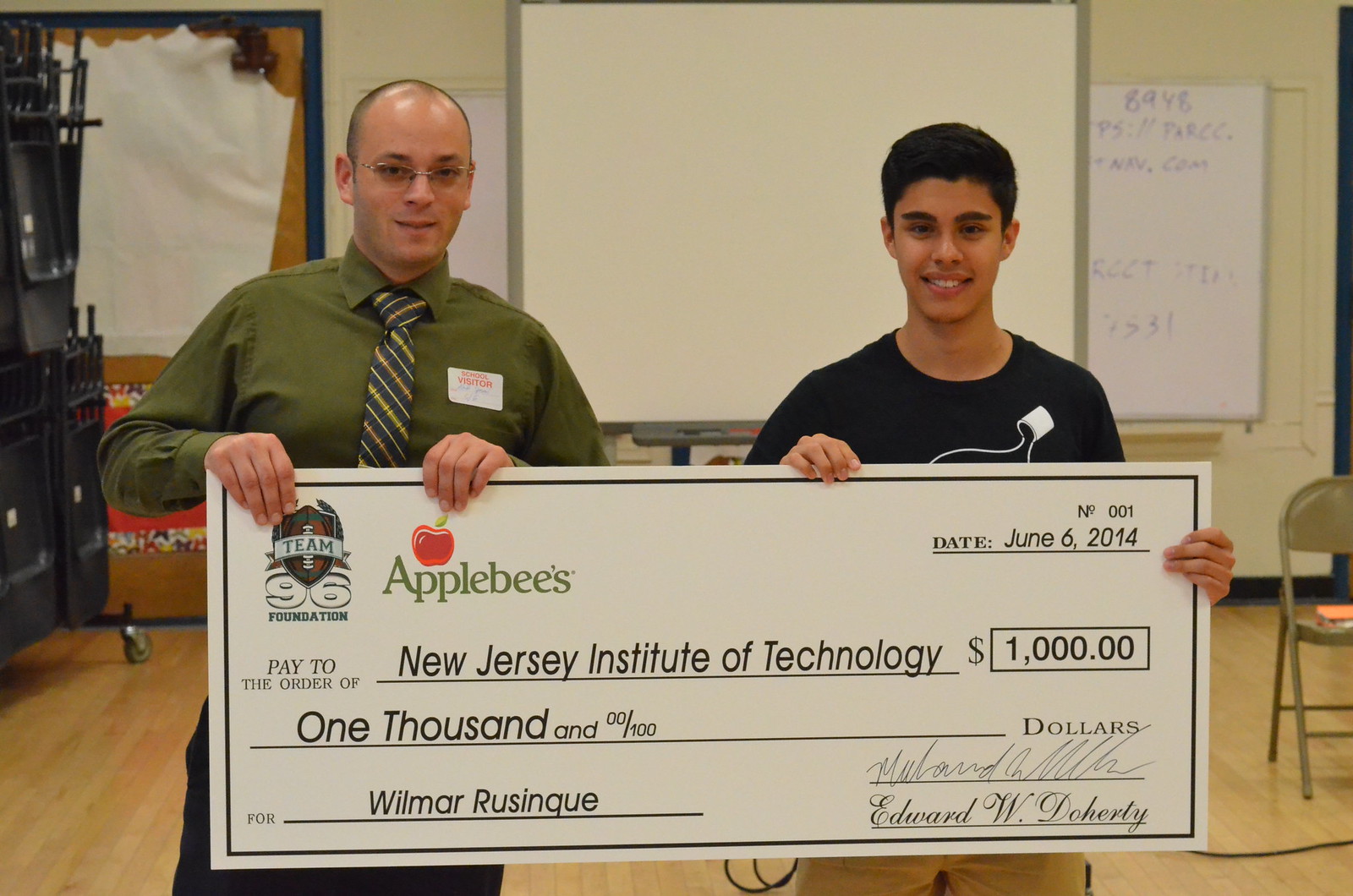The color photograph, in landscape orientation, features a man and a young teenager standing in the center, both facing the viewer and holding a large novelty check. They appear to be in a classroom or similar setting, indicated by the presence of a folded up tables and chairs to the left and a whiteboard with faint writing to the right. The check, adorned with the Applebee's logo and labeled "Team 96 Foundation," is dated June 6th, 2014, and made out to the New Jersey Institute of Technology for the amount of $1,000. The check specifies that the funds are for Wilmar Rusenque, and it bears two signatures, including one from Edward W. Doherty. The man on the left is dressed in a dark olive shirt and tie, and is bald-headed, while the young teenager on the right, possibly around 15 years old, has dark hair and wears a black t-shirt. The photograph encapsulates a moment of financial award and recognition, likely celebrating Wilmar's academic or project achievements.